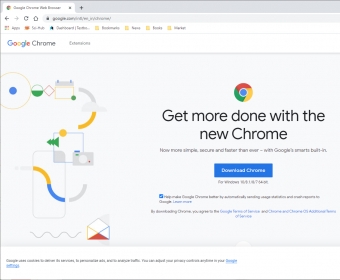This is an image of a Google Chrome promotional webpage. The header prominently displays the recognizable Google Chrome logo with its classic red, blue, green, and yellow colors. Although the text in the search bar is too small to be legible, the webpage is clearly identifiable as related to Google Chrome. On the left-hand side, there is a detailed diagram consisting of geometric shapes and lines: a yellow and blue circle intersect with a green circle, which connects to a red diamond. This network leads to a yellow box and continues through a series of shapes, including a half-gray, half-yellow circle and a green-edged box with a yellow dot inside. This complex arrangement feeds into another box featuring gold and blue colors. Ultimately, the diagram ends with a small, colorful squiggle that leads into an envelope icon outlined in multiple colors with a red section at the bottom. The main text on the webpage reads, "Get more done with the new Chrome" with the Chrome logo above it. Below this headline, there is additional, very small text that is unreadable, but a blue button labeled "Download Chrome" stands out, accompanied by some additional text in black and blue under the button.